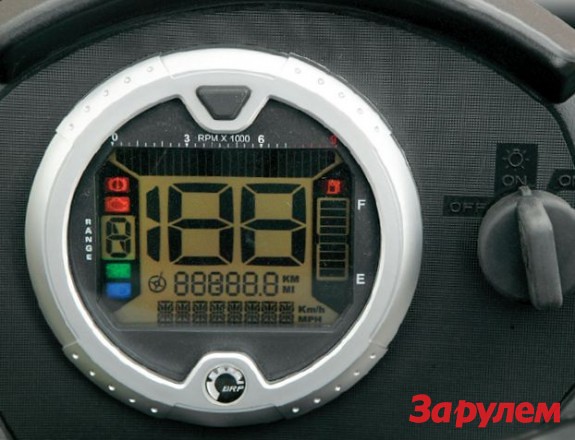This photograph showcases the digital odometer of a vehicle, prominently displaying a reading of "188" for the trip distance, alongside a total mileage of "88888.8." The odometer is set within a round, silver metallic frame, contrasting against the black, slightly arched, and textured dashboard. The digital display window is square with a beige background and black numerical digits. To the immediate right of the odometer, there is a dial with labeled positions for "on" and "off," presumably for controlling the vehicle's lights. The fuel gauge indicates that the tank is empty. A red watermark featuring text in a Cyrillic font is visible in the lower right-hand corner, adding an intriguing, albeit unreadable, detail to the image.